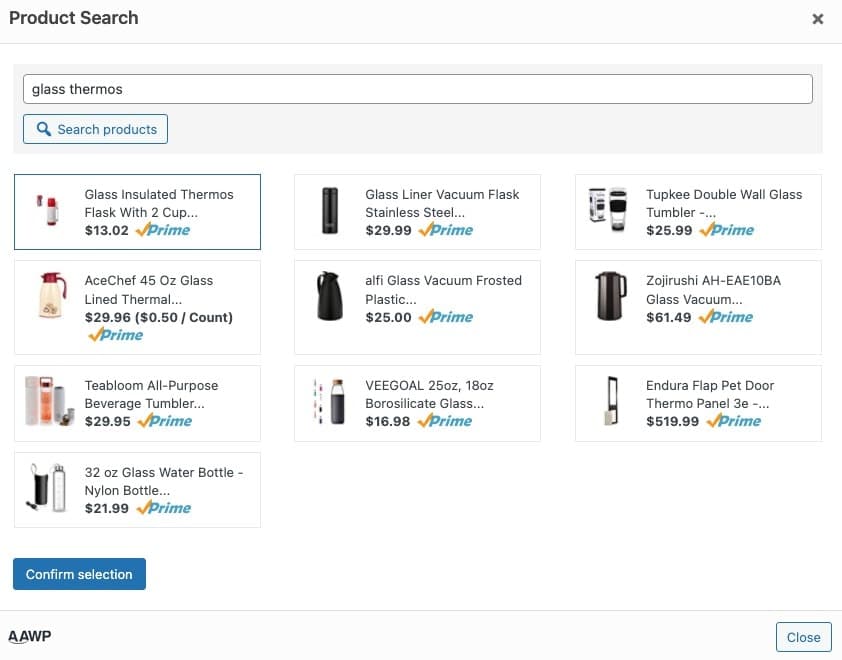**Detailed Caption for Amazon Product Search Screenshot:**

The image is a screenshot of a product search on Amazon, displayed on a clean white background. In the upper left corner, the text "Product Search" is prominently printed in black, accompanied by an "X" symbol to its right which likely serves as a close button.

Directly below this, there is a white search box containing the query "glass thermos" written in black letters. Adjacent to the search box, a blue button marked "Search Products," featuring a small magnifying glass icon, invites users to initiate the search.

Beneath the search interface, a series of rectangular boxes spans from left to right, each representing a different product. The first box, highlighted with a blue outline, displays a product called "Glass Insulated Thermos Flask with Two Cups" and shows its price as $13.02, accompanied by the Amazon Prime icon.

Following this, other product options are listed as follows:

1. **Glass Liner Vacuum Flask Stainless Steel** - $29.99 (Prime)
2. **Tupe Key Double Walled Glass Tumbler** - $25.99 (Prime)
3. **Ace Chef 45 Ounce Glass Lined Thermal** - $29.96 (50 cents per count, Prime)
4. **Alfie Glass Vacuum Frosted Plastic** - $25.00 (Prime)
5. **Zoe Rishi AH-EAE10BA Glass Vacuum** - $61.49 (Prime)
6. **Tea Bloom All-Purpose Beverage Tumbler** - $29.95 (Prime)
7. **Vgold 25 Ounce, 18 Ounce Borosilicate Glass** - $16.98 (Prime)
8. **Endura Flap Pet Door Thermal Panel 3E** - $519.99 (Prime)
9. **32 Ounce Glass Water Bottle, Nylon Bottle** - $21.99 (Prime)

Each product is accompanied by a corresponding icon image to the left of its description.

At the bottom of the search results, a blue button labeled "Confirm Selection" in white text stands ready for user interaction. Lower down, there are two options: "A-A-W-P" on the left, and another blue button marked "Close" on the right.

This organized layout allows for easy browsing and selection of various glass thermos products available on Amazon.